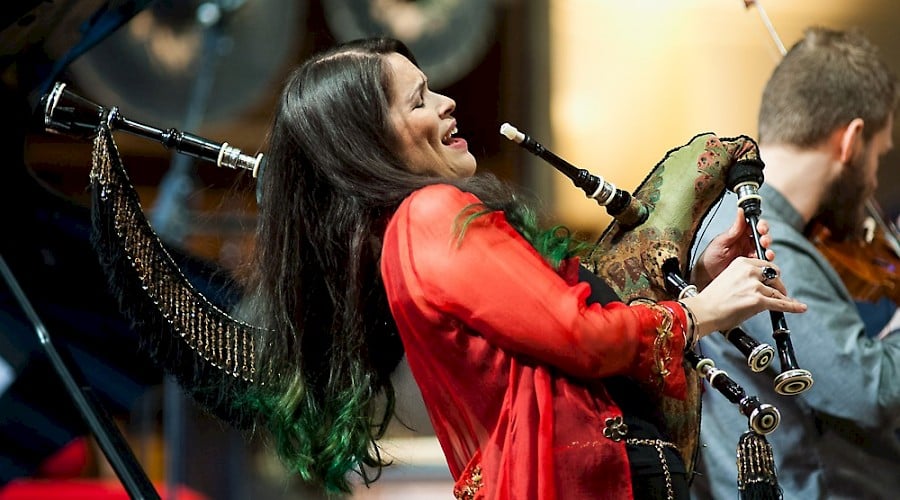In this professionally taken close-up photo of a band in performance, two musicians are deeply engaged in playing their instruments. At the center, a woman in a vibrant, sheer red silk top, with long black hair featuring green tips, passionately plays a unique wind instrument that resembles a bagpipe with multiple pipes and reeds. Her eyes are closed, and she appears to be enjoying the moment, possibly singing. Beside her, a man with light brown hair and a beard is absorbed in playing a brown wooden violin. He is dressed in a blue long-sleeved shirt. Both musicians are in dynamic motion against a fully blurred background, highlighting the intensity and emotion of their performance.